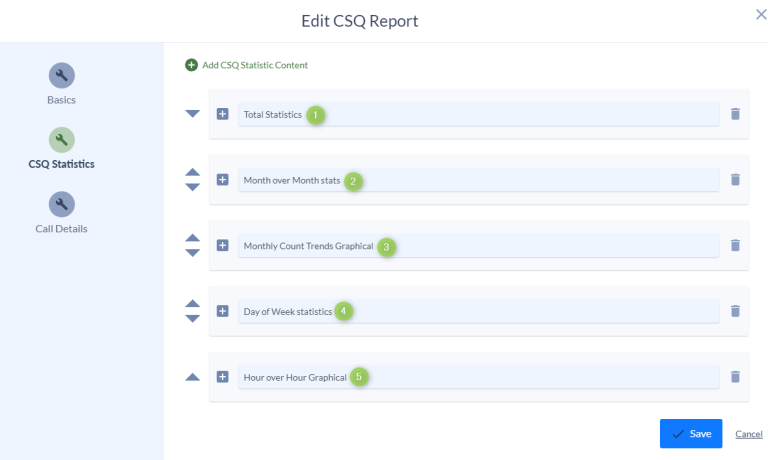The image depicts an analytics page with various statistical insights. On the left side, there is a very pale blue sidebar featuring three identical wrench icons. Each icon directs the user to a different page: "Basics" at the top, "CSQ Statistics" in the middle, and "Call Details" at the bottom. Currently, the "CSQ Statistics" page is selected. At the top of the main content area, a white header with dark grey text reads "Edit CSQ Report." Below this header, the main page, which has a white background with grey and blue text boxes, includes a green text heading that says "Add CSQ Statistic Content." Following this heading, there is a row of blue rectangular boxes, each dedicated to different functions related to CSQ statistics. In the very lower right-hand corner, there are two buttons: "Save," displayed in white text on a blue background, and "Cancel."